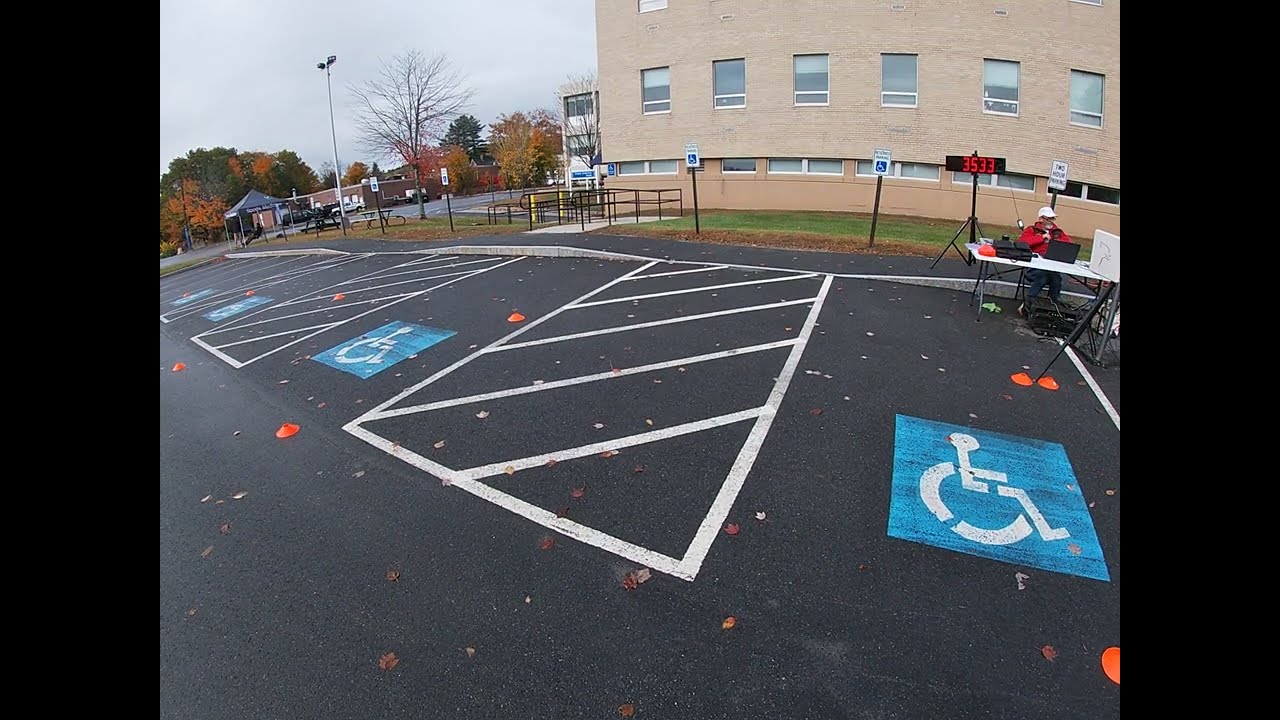The image depicts a daytime scene in a parking lot in front of a multi-story brown brick building. The asphalt ground, adorned with white lines, primarily serves several handicapped parking spaces, each marked with a blue square logo featuring a person in a wheelchair. Adjacent to the left of these blue logos, there are white rectangular shapes with diagonal white stripes painted on the ground.

In the upper right part of the image, a man in a red coat and white hat sits at a white table set up in one of the handicapped parking spaces. He appears to be working on a laptop, with two black bags on the table beside him. Behind him stands an electronic sign displaying the number 3533 in red.

The scene includes additional details such as a gray sky overhead, a patch of grass accompanied by a railing and sidewalk, and a tent in the upper left corner. There are benches, a canopy, and trees in varying autumn colors—red, yellow, and green, including one bare tree. In the distant background, another building and more trees complete the picturesque setting.